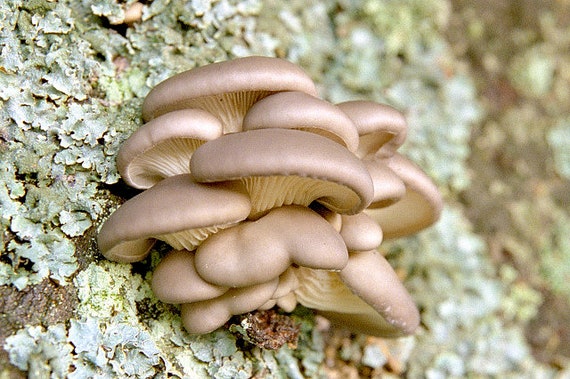This close-up photograph captures a stunning cluster of pearly gray, oyster-like mushrooms with pristine white gills, numbering between eight to twelve. They are growing out of a tree adorned with lichen and old moss. The mushrooms, also called shelf mushrooms due to their stacked formation, appear exceptionally clean and shiny, suggesting their professional presentation. The tree bark, covered with lichen and moss, serves as the textured backdrop, which is slightly blurred to enhance the mushrooms' sharp foreground focus. This detailed and clear image, likely taken by a skilled photographer or mycologist, emphasizes the organic beauty of the scene. The vibrant mushrooms contrast beautifully against the muted tones of the mossy tree bark, creating an exquisite nature study.